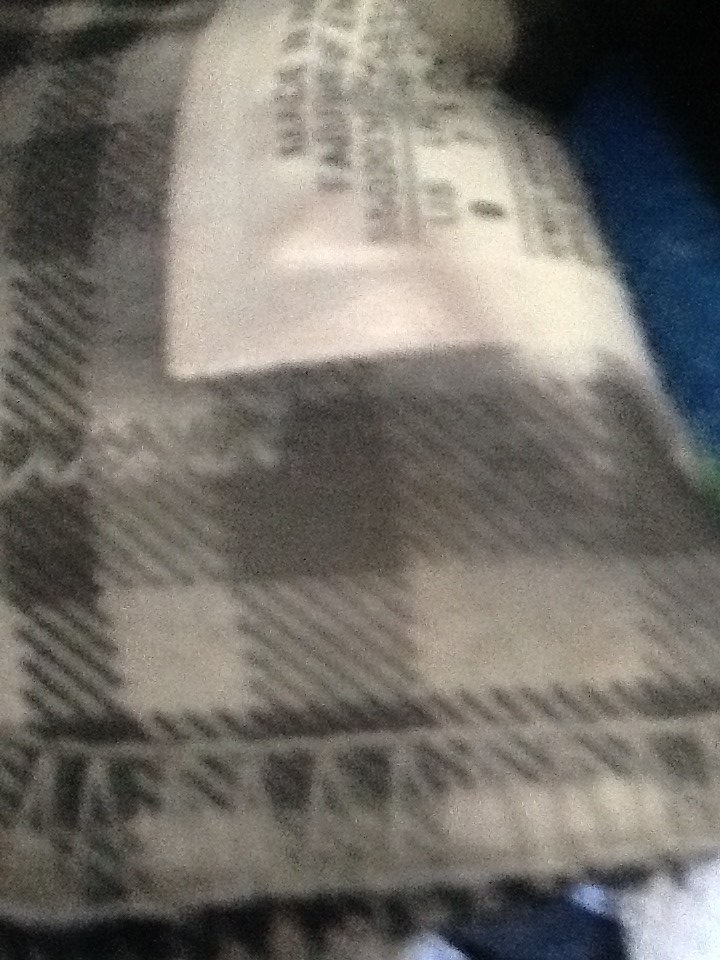This photograph features a close-up view of a flannel plaid fabric, possibly part of a blanket or shirt. The fabric displays a muted color palette consisting of gray, beige, and black tones. The image is notably blurry, making it difficult to discern fine details. Prominently visible is an off-white tag with black lettering, but the text remains unreadable due to the blurriness. The presence of the tag, along with visible stitching and seams, suggests that this is the interior side of the fabric, likely where the edge was folded and sewn. The composition lacks additional elements, such as text or other objects, that could offer further context or help identify the exact item.